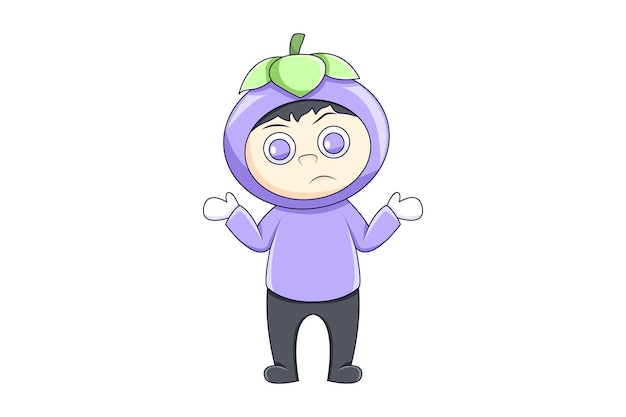The image is a detailed cartoon drawing of a small child-like character on a plain white background. The character, who has light skin and black hair peeking out from under a peculiar headpiece, appears to be wearing a costume. The headpiece resembles a purple berry with a hole where the child's face is visible. At the top of the berry, there are three green leaves and a stem. The child has large, blue eyes, and a frowning, quizzical expression as if saying, "I don't know." He is dressed in a light purple shirt, gray pants that blend seamlessly into his feet, giving the impression that he has no shoes. His arms are extended outwards, and he is wearing white mittens, adding to his curious and whimsical appearance.